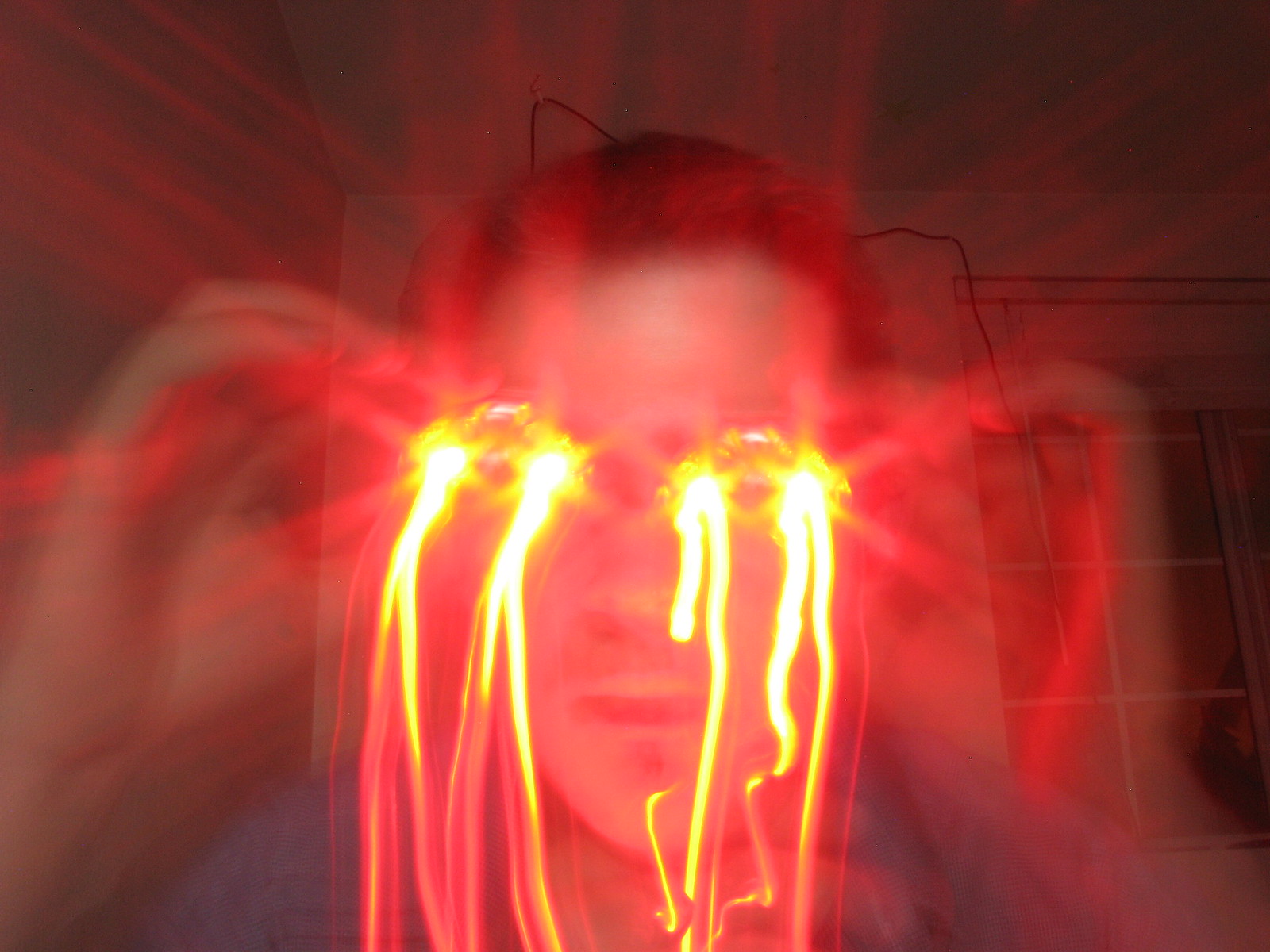The image depicts a heavily blurred and dark scene dominated by rich red hues. At its center is a figure, likely a man, whose features—including the outline of his face and hands—are subtly discernible through the blur. He appears to be wearing glasses, each lens fixed with two small lights. These lights, positioned one on each side of the lens, create intense, eye-catching trails as they seem to move. The movement or shaking of these glasses has produced striking light artifacts, creating a spectacle of vibrant red and intense yellow streaks that resemble waterfalls or dripping light. These streaks emanate from the figure's eyes and cascade downward, transitioning from bright yellows to deep oranges, contributing to a dramatic and surreal visual effect. The overall impression is one of a dreamy or otherworldly light painting, where the beauty of light and motion is captured in a single mesmerizing shot.